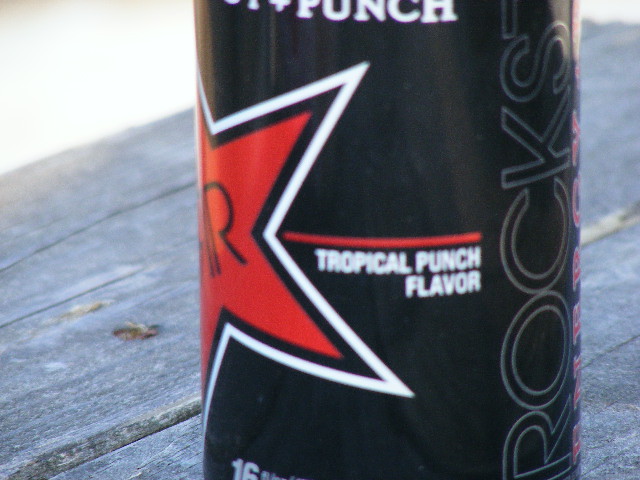This close-up image features a black can, cropped at the top and bottom, rendering it partially obscured and difficult to identify fully. At the top of the can, the visible letters spell out "P-U-N-C-H" and a red star outlined in white and black prominently stands out. Inside the star, black letters are partially visible with an "R" discernible. To the right, a red line is observed just above the white text, which reads "tropical punch flavor." Near the bottom, the number "16" can be seen, suggesting it is a 16-ounce can. Along the side of the can, the word "R-O-C-K-S" is written vertically but is incomplete. The can rests on a gray wooden table or counter, with a white background providing contrast.